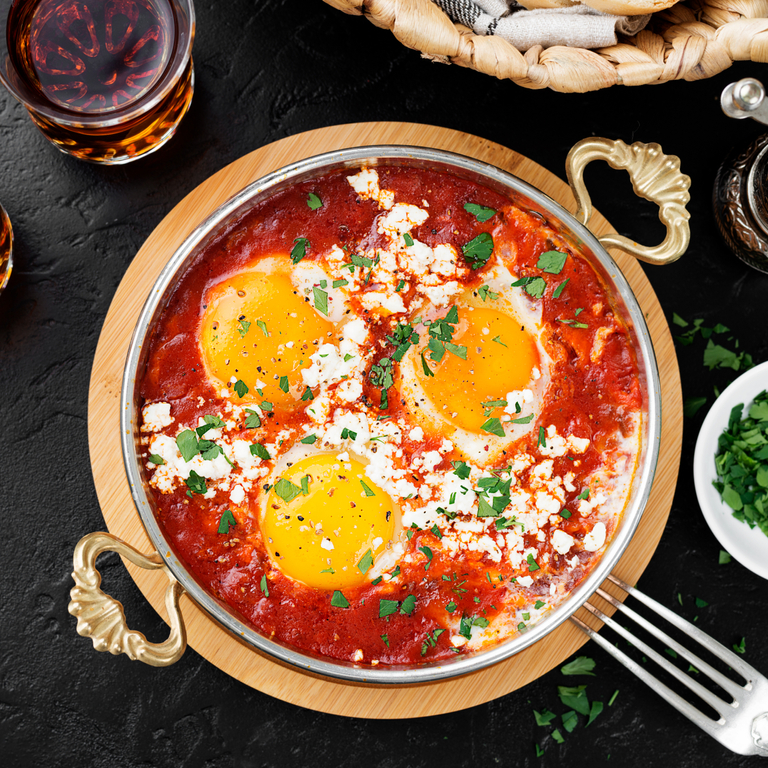The image captures a professionally shot, detailed close-up of a high-end Turkish breakfast spread, prominently featuring a dish of menemen. The scene is carefully lit and sharply in focus, making it suitable for advertisement in magazines or on social media. At the heart of the composition is a round, ornate bowl with gold handles, resting on a wooden base. The bowl contains three vibrant yellow egg yolks nestled in a rich red marinara sauce, sprinkled with white cheese, possibly feta, and dotted with green herbs such as cilantro or parsley.

Surrounding the main dish, the black textured table holds a variety of elements that add to the sophistication of the setting. In the lower right corner, a shiny silver fork lies next to a small white dish filled with chopped greens, likely cilantro or basil. The upper portion of the image reveals part of a wicker bread basket, partially covered by a napkin, hinting at fresh bread inside. To the left of the basket sits a clear glass filled with a brown liquid, possibly iced tea. The harmonious arrangement of colors—yellow, red, white, green, and brown—along with the luxurious touches, suggests this photograph was taken at an upscale restaurant and conveys a sumptuous dining experience.